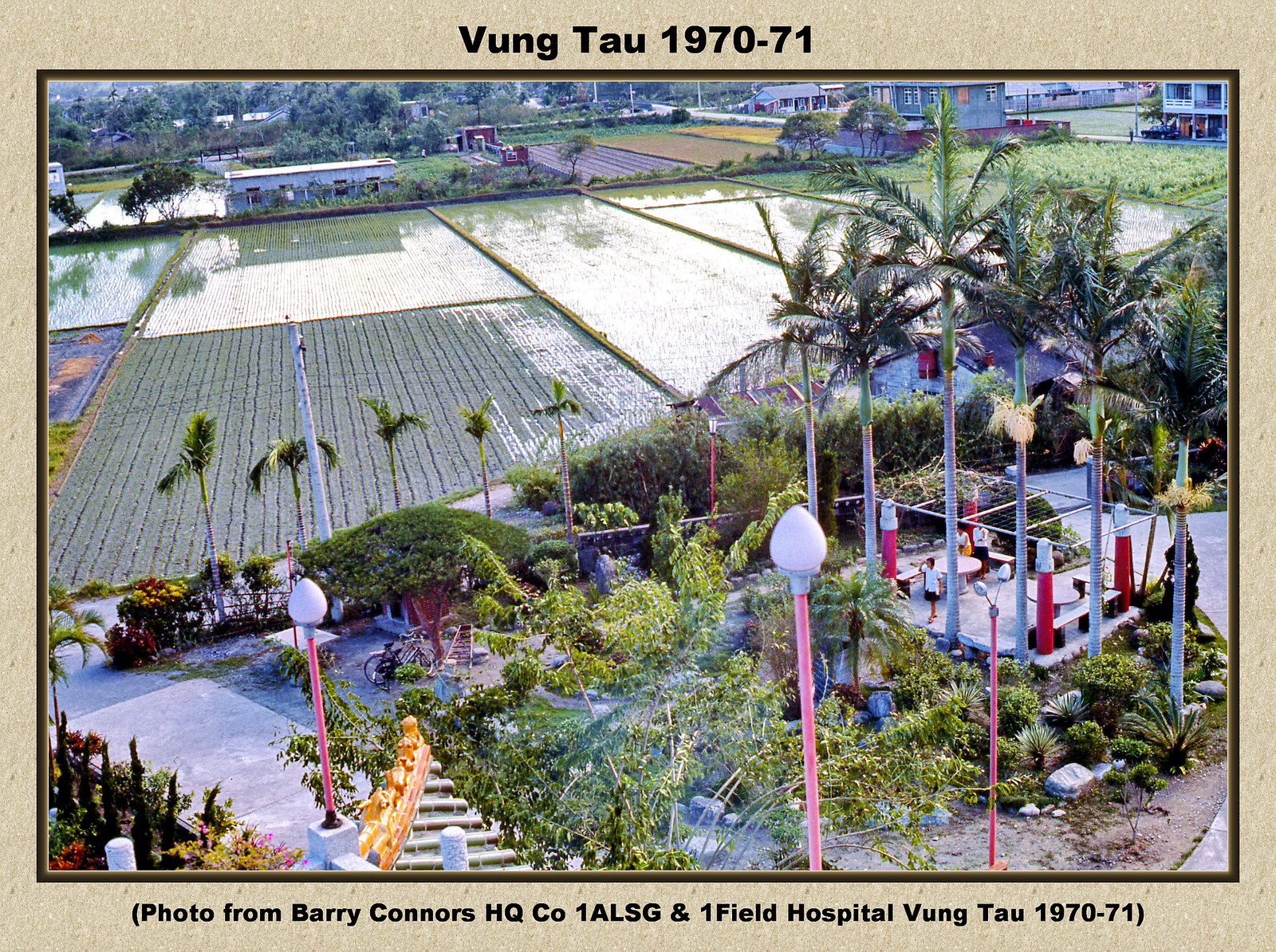This is a photograph labeled "Vu Tau 1970-71" at the top and "Photo from Barry Connors HQCO 1ALSG and 1 Field Hospital Vu Tau 1970-71" at the bottom. The image depicts a landscape with sectioned fields, likely rice paddies, filled with water. In the foreground, there is a garden area with palm trees, light posts, and some paved, cemented sections, possibly a stone walkway. The garden appears to include tables and a setup resembling a picnic area, indicating a park-like environment within the field backdrop. Scattered throughout the scene are various types of vegetation planted in organized rows, suggesting a farm-like setting. Trees and bushes frame the composition, and some people are visible in the distance, adding life to this tranquil yet industrious landscape.